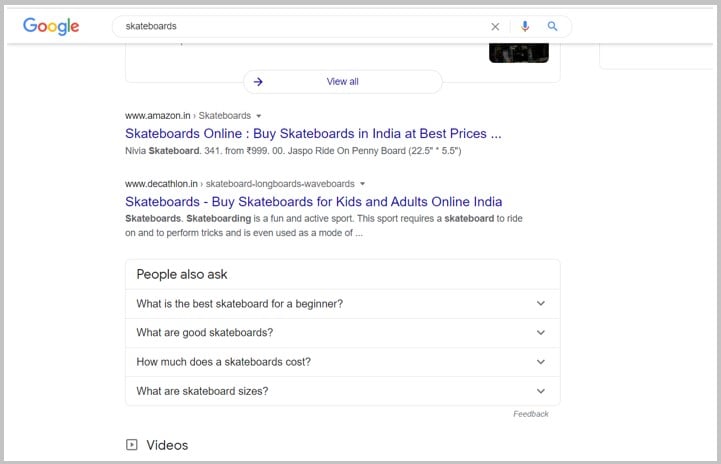The image displays a Google search results page with the search term "skateboard" entered in the search bar. Prominently featured on the top left is the Google logo. Below the search bar, various search results are listed. The first search result suggests "skateboard online" with a hyperlink to buy skateboards in India at the best prices from Amazon's Indian website (www.amazon.in). The second search result is from Decathlon India (www.decathlon.in), offering a variety of skateboards for both kids and adults under the link "skateboards-longboards-withboards."

Additional elements in the search results include descriptions highlighting that skateboarding is a fun and active sport, requiring a skateboard for riding and performing tricks. It is also noted that skateboards are used as a mode of transportation. There are prompts for frequently asked questions such as, "What is the best skateboard for a beginner?", "What are good skateboards?", "How much does a skateboard cost?", and "What are skateboard sizes?". These details provide an overview of the various considerations for potential skateboard buyers and enthusiasts.